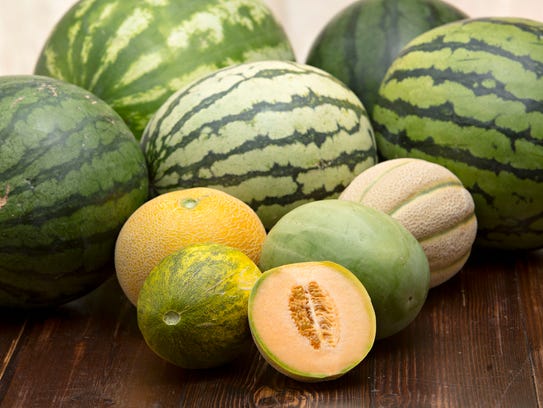In this vibrant color photograph, various melons are artfully arranged on a rich, grainy, dark brown wooden table, set against a white wall. The composition includes a mix of five large watermelons at the back, all displaying distinctive patterns of light green and dark green striations in varying shades and sizes. The largest watermelon, situated towards the back, is a unique green and tan color. Two other watermelons feature darker green stripes, while one on the far right showcases a lighter green hue with notable dark stripes. The center watermelon stands out as the lightest, adorned with dark stripes. 

In addition to the watermelons, several other melons are present. Prominently, a sliced cantaloupe in the middle reveals its light orange interior and a couple of rows of thick seeds. To the left front, we see another green and yellow splotched melon, resembling a cantaloupe, while behind it, a honeydew-like melon adds variation to the scene. The array of melons, transitioning from smaller in the front to larger in the back, creates a visually appealing gradient of color and size, highlighting the diversity among the melons displayed.